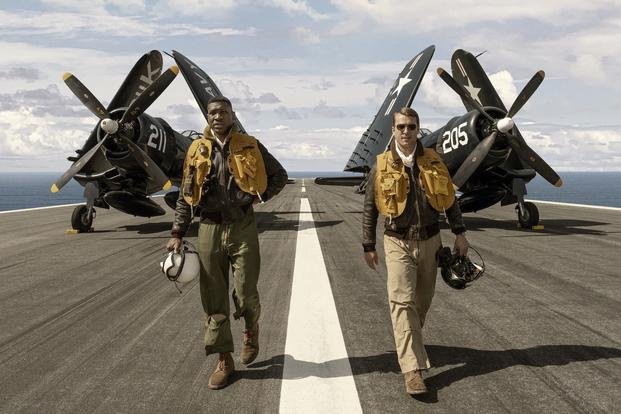The image captures two World War II aviators walking away from their aircraft on the deck of an aircraft carrier, set against a backdrop of an overcast sky and a calm sea. Both planes on the runway are military green, with the one on the left featuring the identifier '2-1-1' on its engine cowl, likely confirming it as a Bedouin Gulf F4U Corsair. The plane on the right also appears to be a Corsair, inferred from its folded wings and propeller size, showing the number '205' and a star on its wings. The runway itself is a dark grayish-brown with a distinct white line running down the center.

The pilot on the left is an African American dressed in dark brown trousers, brown shoes, and a dark brown shirt with a yellowy brown vest over it. He sports an olive drab flight suit and a dark brown or black leather jacket, and he carries a white helmet trimmed in brown in his right hand. The pilot on the right is Caucasian, wearing light khaki pants, brown shoes, a beige scarf, dark brown leather jacket, and a similar yellowy-brown vest. He has light brown hair, wears aviator sunglasses, and holds his helmet in his left hand. The evident camaraderie and history between the two pilots make this a compelling capture of World War II aviation.